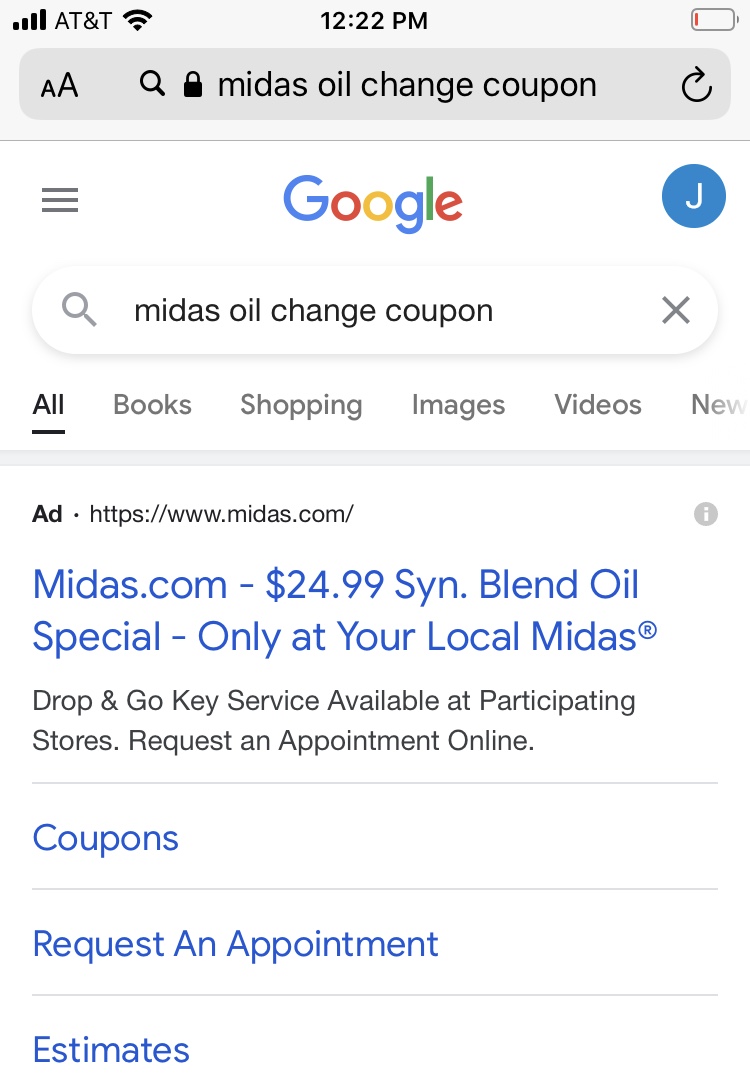The image displays a screenshot of a smartphone screen. At the top, the status bar shows the AT&T network, signal strength bars, a Wi-Fi symbol, the time "12:22 PM", and the battery percentage. Below this is a gray search box containing the text "Midas Oil Change Coupon" along with a magnifying glass icon, a lock icon, and a refresh circle symbol.

The main part of the screen features a Google search results page. At the top left is the colorful Google logo, and next to it is a profile icon with the letter "J" on a blue background. In the Google search bar, the text "Midas Oil Change Coupon" is also displayed, with a gray 'X' and a gray magnifying glass icon.

The search results page is divided into sections: All, Books, Shopping, Images, Videos, and News. At the top of the search results is an advertisement. The ad's URL "HTTPS://www.midas.com" is displayed prominently, along with a gray information icon ('i'). The ad text reads: "Midas.com $24.99 Sin Blend Oil Special, only at your local Midas" in blue text. Additional information in black text states, "Drop and Go Key Service available at participating stores. Request an appointment online."

The ad also features three blue buttons labeled "Coupons," "Request an Appointment," and "Estimates." The background of the screen is primarily white, with the gray Google search bar remaining fixed at the very top.